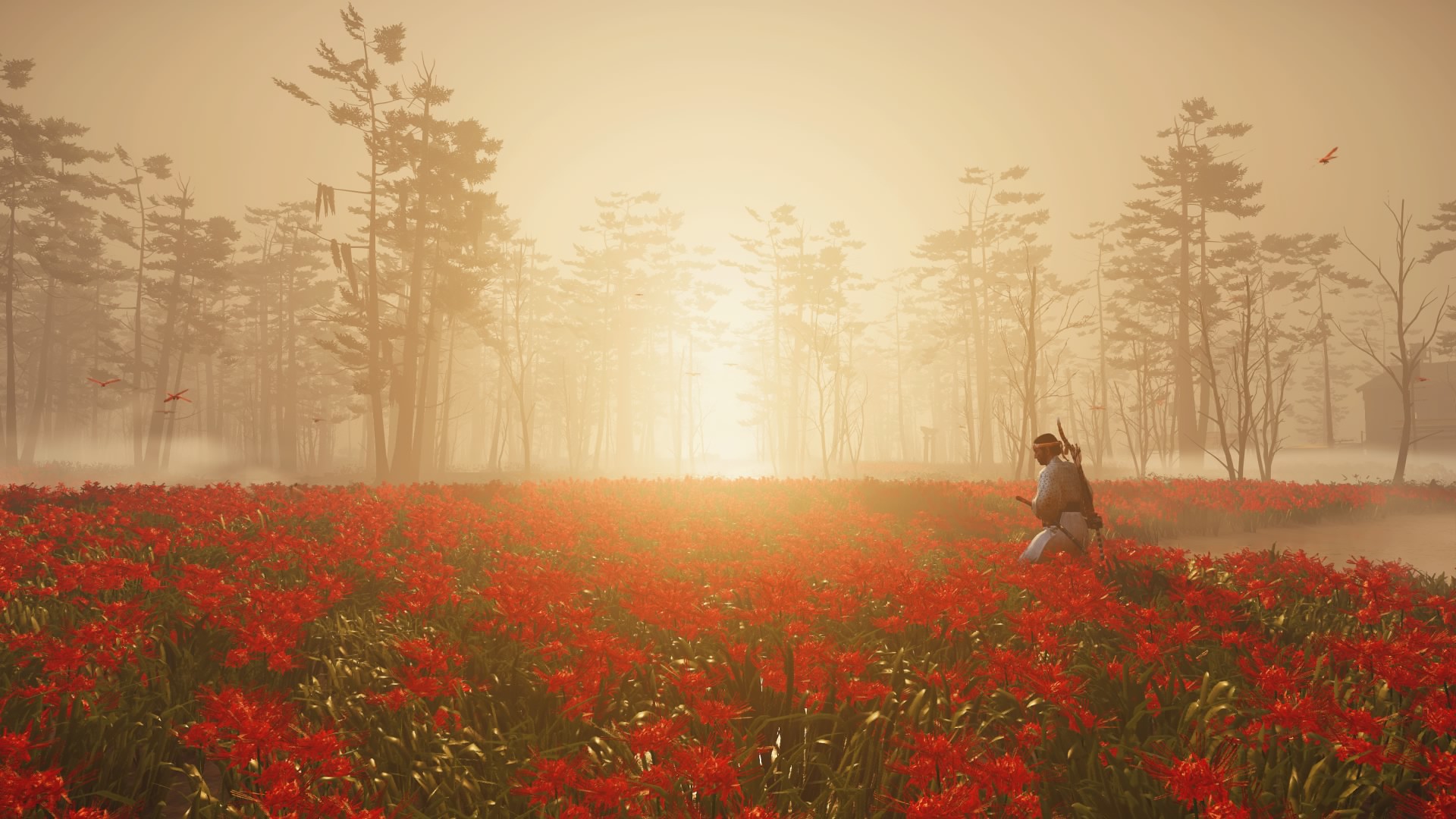In this scene, which could either be from a video game or a piece of digital art, a character stands amidst a vast field of red flowers. Positioned just to the right of the center, the character is neither in the foreground nor the distant background, appearing approximately 20 to 30 feet from the viewer's perspective. Clad in a white robe-style garment and wearing a headband, the character wields a curved sword, reminiscent of a samurai katana, and carries a bow with arrows slung over their back. The setting suggests an early morning ambiance, as a low fog blankets the background, giving way to the silhouettes of trees stretching across the scene from left to right. The mist is softly illuminated by the rising sun, casting a gentle light over the serene landscape.